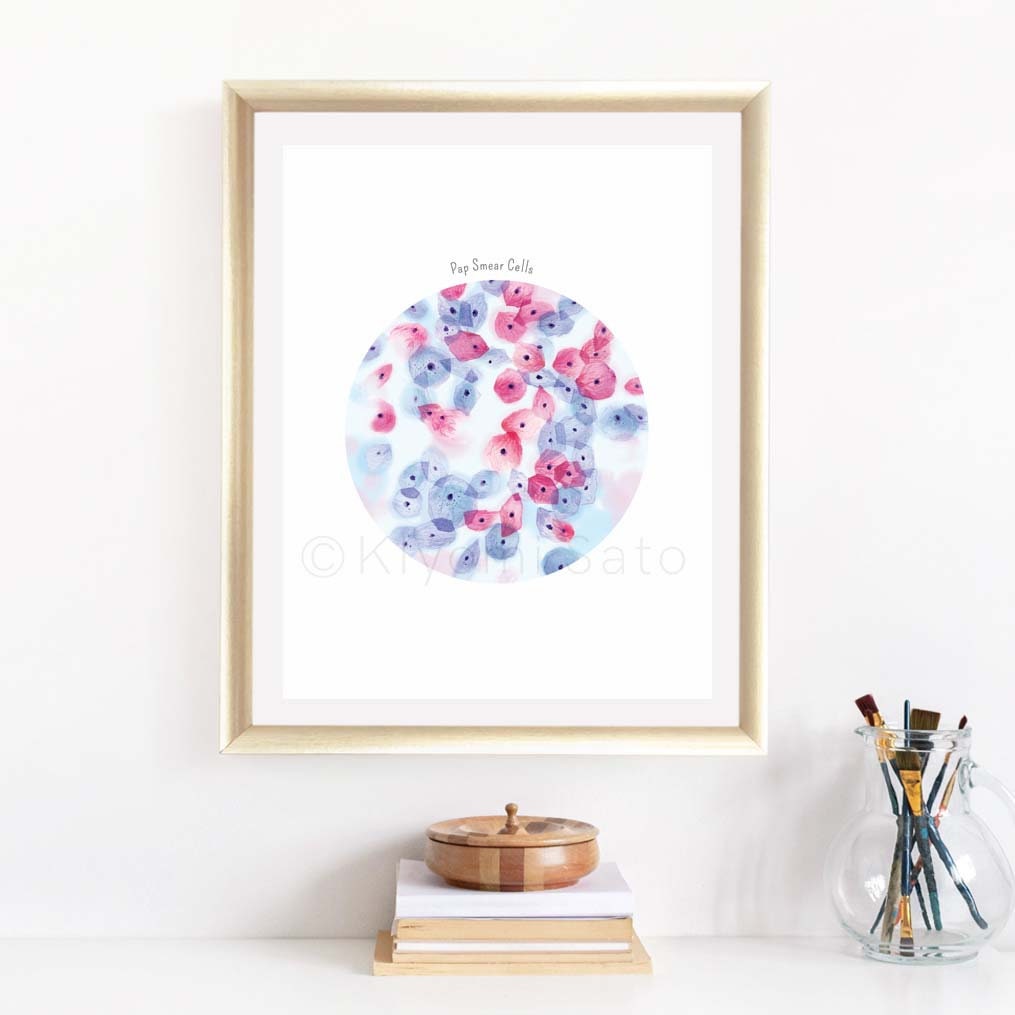The image is a vertical, rectangular photograph of a picture hanging on a white wall. The picture is framed with a brown frame and features a white matting. The artwork within the frame is labeled "Pap Smear Cells." Below this label, there is a large circular section containing various cells depicted in red and blue, each punctuated with small black dots at their centers. Overlaid on the image is a watermark featuring a symbol and the name "Kai Sato," though the text is somewhat difficult to read. The scene also includes a white countertop situated beneath the picture. The countertop holds several beige and white books, alongside a small, lidded container that appears to be made of wood. On the right side of the countertop stands a vessel filled with paintbrushes.